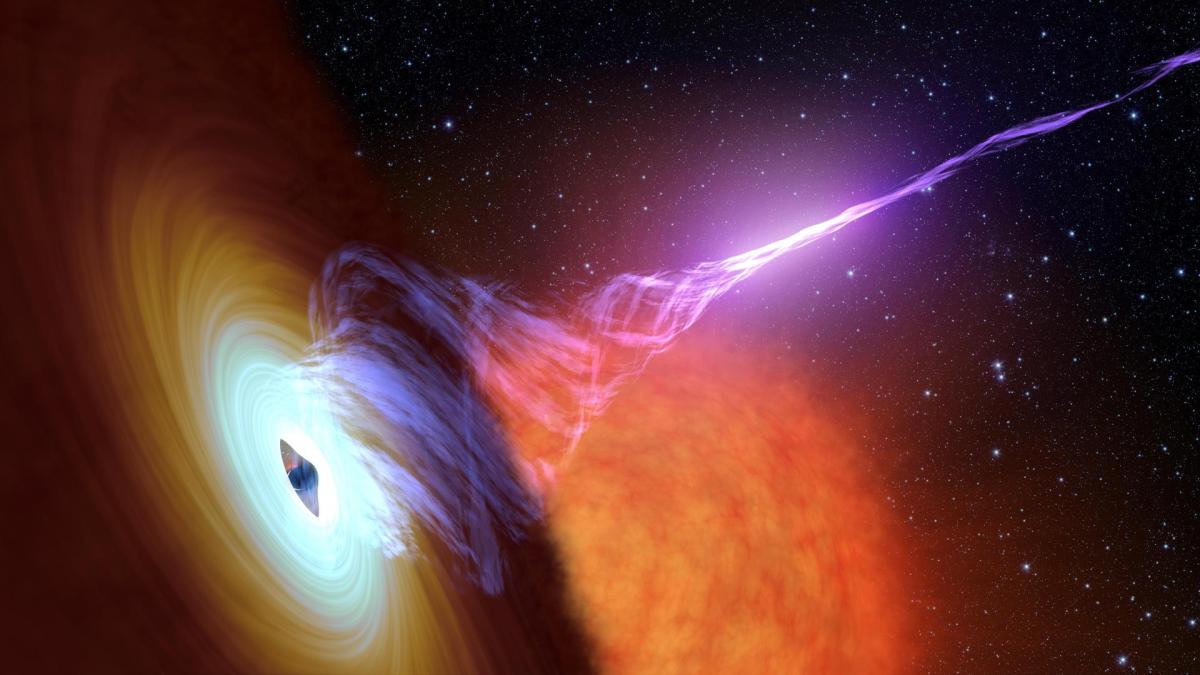The image portrays a highly detailed representation of an astronomical phenomenon, likely depicting a black hole or an artistic interpretation thereof. On the left side of the image, a swirling maelstrom of colors transitions from deep reds to oranges, then to yellows, and finally converges into a bright white center resembling the typical appearance of a galaxy or a spiral nebula. Dominating the center is a dark, eyeball-shaped depression flanked by the intense white light, suggesting the black hole's event horizon where matter is being inexorably drawn in by gravitational forces.

Emerging from the central white swirl, there is an intriguing object with a spaceship-like silhouette, surrounded by a mix of the same swirling universe colors. From this object, a purplish streak of light extends upwards, resembling a tornado of luminescence, and stretches to the upper right corner, intensifying into a laser-like beam. 

Beneath this celestial ballet is a pronounced orange burst, resembling a cloud or a flaming ball, which sets off the more vivid elements against the dark expanse of space. The background is punctuated by numerous stars, adding depth to the cosmic scene. The abstract blend of light and dark hues, along with the intricate details, vividly captures the otherworldly nature of such an interstellar event.